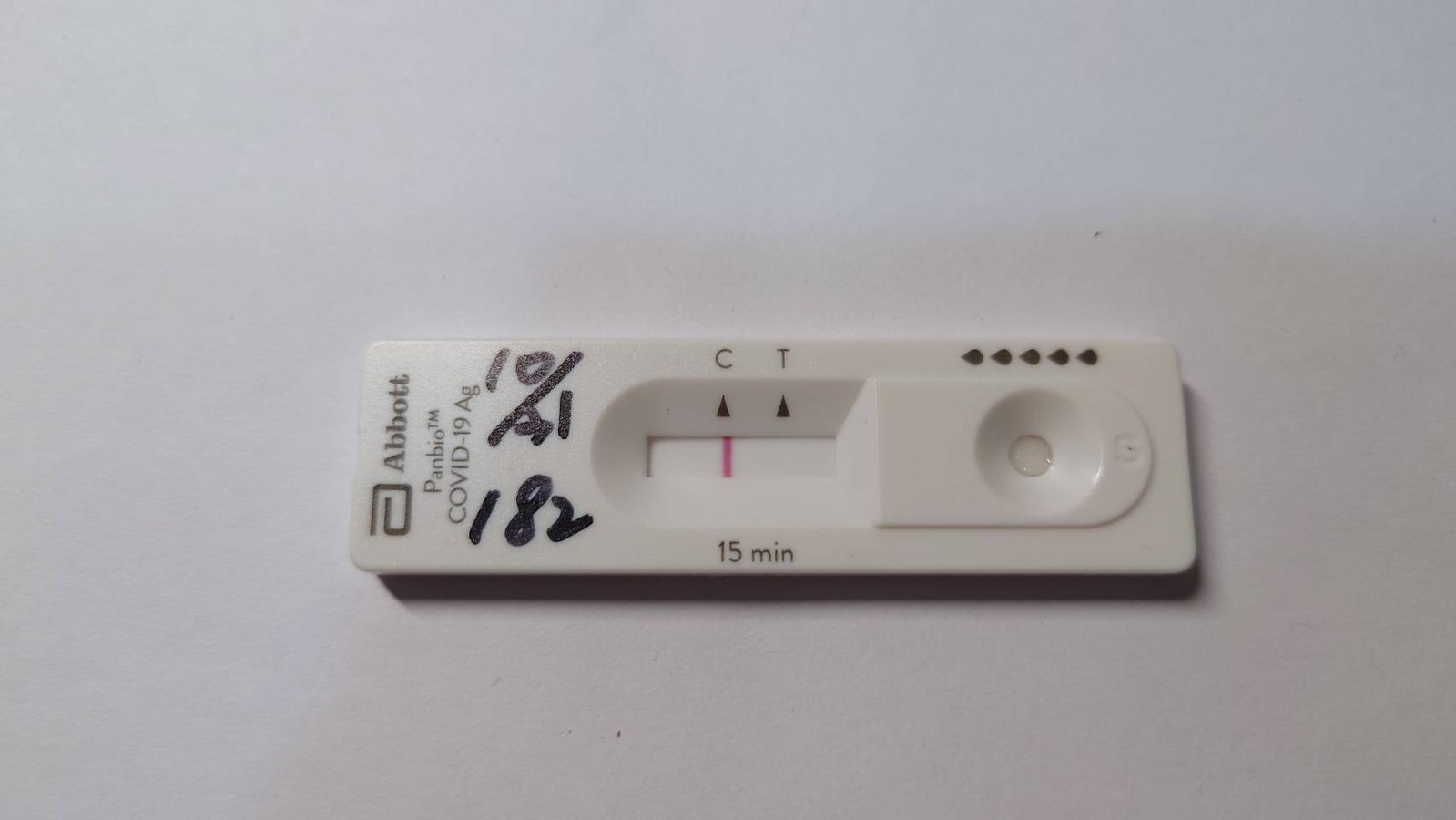This color photograph showcases a COVID-19 rapid antigen test, manufactured by Abbott Laboratories. The plastic test strip, rectangular in shape, is placed horizontally. The top portion of the strip bears the Abbott logo and the name 'Abbott' prominently. Directly beneath this branding, the label "COVID-19 AG" indicates it is a rapid antigen test.

Handwritten with black marker, several numbers are visible on the strip: '10/41' appears on the left side, followed by '182' below it. Central to the strip, there's a small window displaying red lines next to the letters 'C' and 'T', which are common indicators for control and test lines in such diagnostics. On the opposite side, "15 MIN" denotes the recommended interpretation time of 15 minutes.

In the upper right corner, six teardrop-shaped dots are visible, accompanied by a circular indentation alongside, completing the detailed design of the test strip.